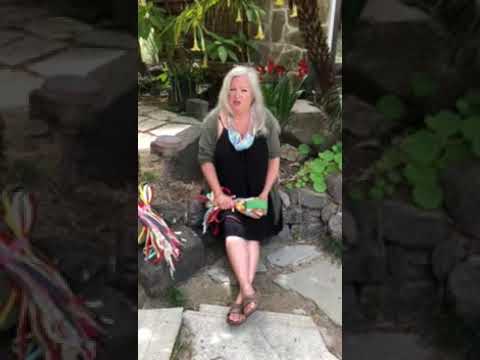In this outdoor image, a white woman in her late 40s or 50s is prominently featured sitting on a low stone wall amidst a garden filled with vibrant tropical plants and flowers. She has medium-length gray hair and is dressed in a dark black dress beneath a gray cardigan, complemented by gray flip flops on her bare feet. The woman, who appears slightly overweight, is looking up at the camera while holding a colorful item featuring green, yellow, and red hues. In the backdrop, the gray flagstones of the garden are visible alongside the trunk of a palm tree, red flowers, and lush green plants, enhancing the tropical ambiance. The scene is illuminated by daylight, accentuating the various shades of gray, black, and colors present in the image.